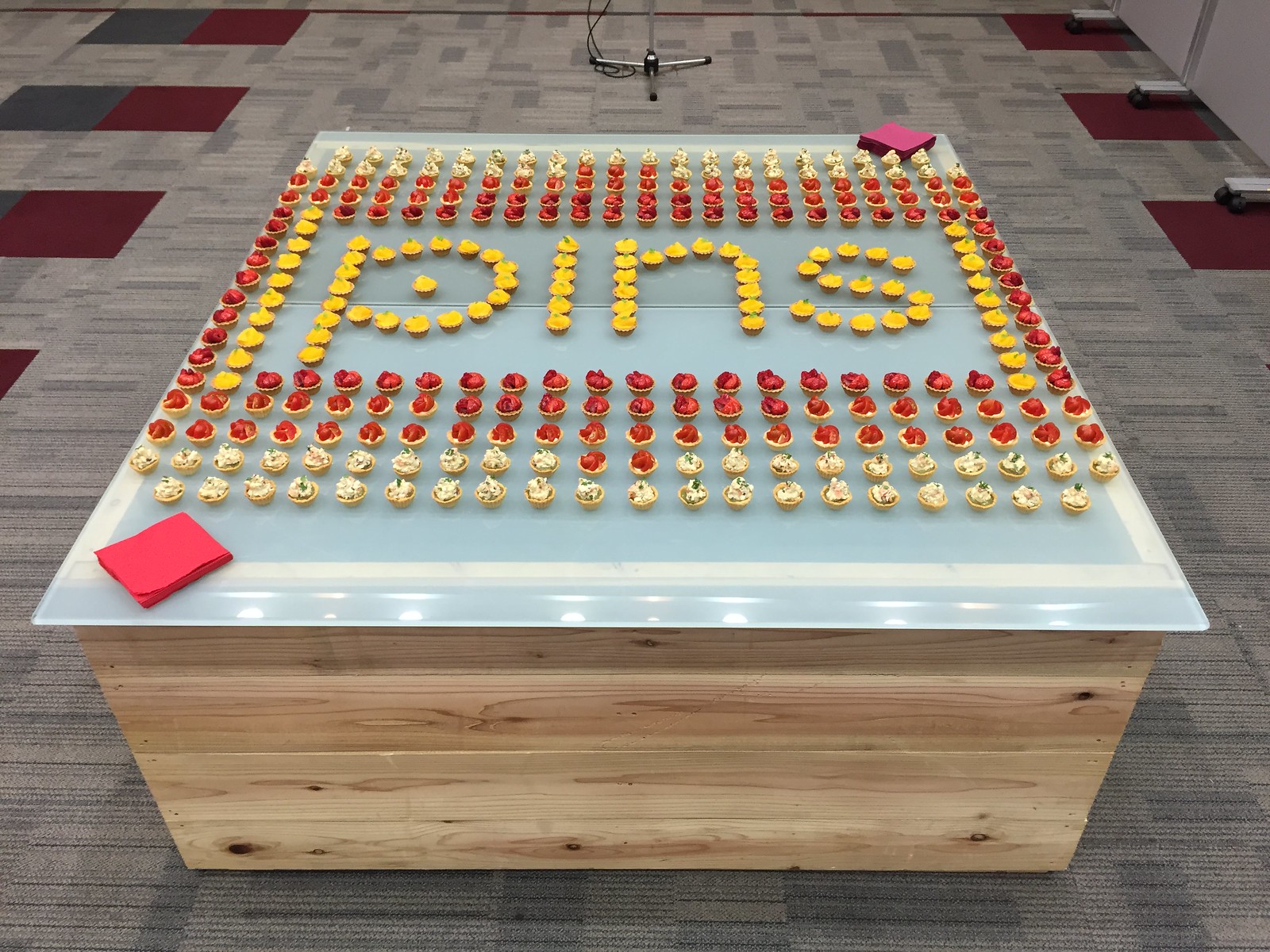In a brightly lit, rectangular office room characterized by short-pile gray carpet and partial cubicle dividers on the right, a large rectangular table stands prominently as the central focus. The table, constructed with a solid base of light, unfinished wood and topped with a slightly translucent, cloudy sheet, possibly plexiglass, supports an intricate display of baked goods, which could be cupcakes or tarts. Arranged meticulously in a square perimeter, the outermost layer consists of white cupcakes, followed by an inner layer of red cupcakes. At the center, yellow cupcakes spell out the word "PINS" within the square formation. Additionally, red napkins are neatly stacked on the bottom left and top right corners of the table, suggesting readiness for consumption. The ceiling features a speaker, enhancing the office atmosphere.